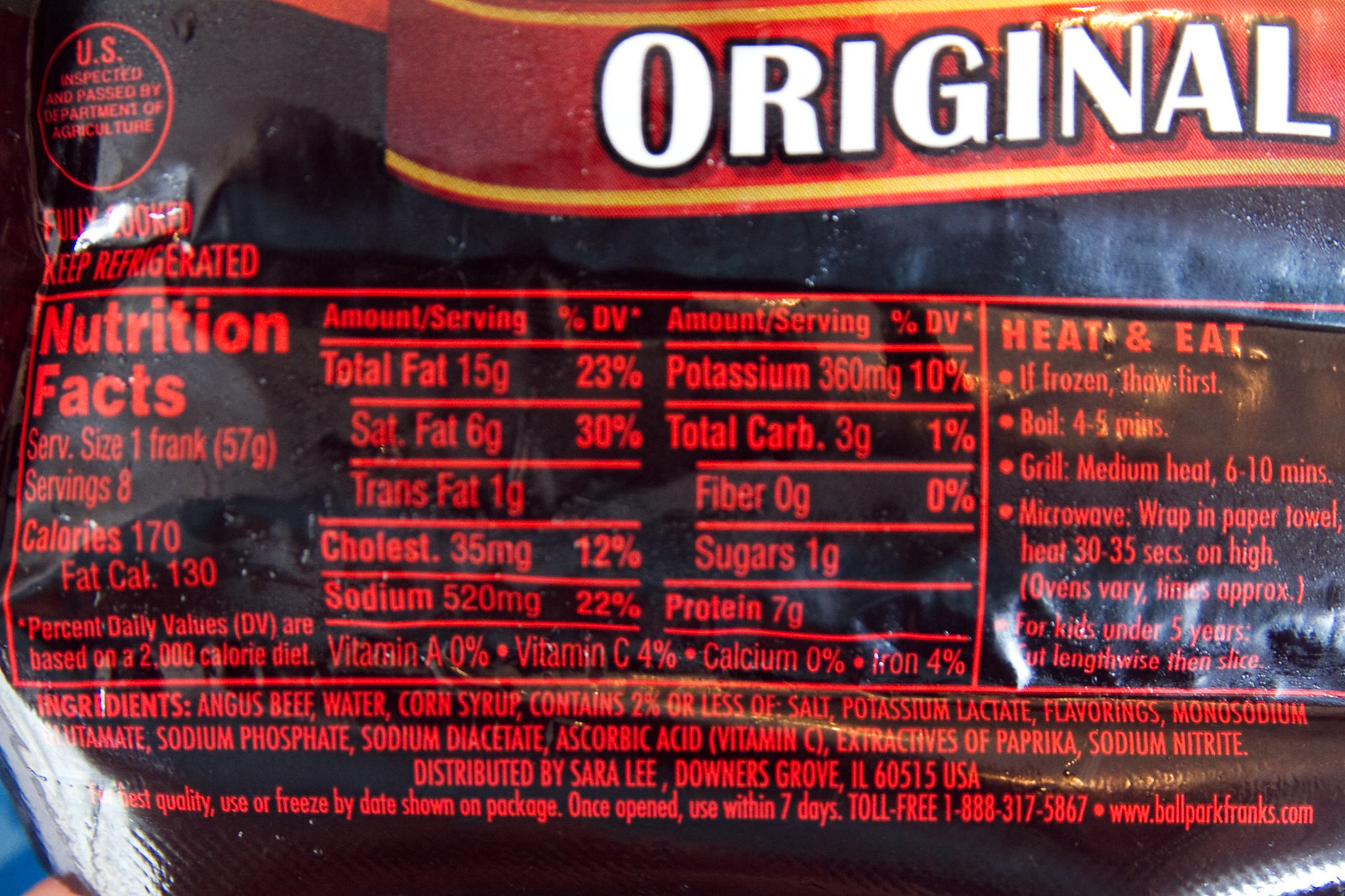The image depicts a detailed Nutrition Facts label for original hot dog franks, distributed by Sara Lee, Downers Grove, Illinois. The package features a logo with the word "original" prominently displayed. A red bubble in the top left corner indicates that the product is "U.S. inspected and passed by the Department of Agriculture." Below this bubble, the text states "fully cooked, keep refrigerated."

The Nutrition Facts panel lists the serving size as one frank (57 grams) with eight servings per package. Each frank contains 170 calories, with 130 of those being fat calories, total fat 15 grams, and saturated fat 6 grams. The product also has a high sodium content with 520 milligrams per serving. Key ingredients include angus beef, water, corn syrup, salt, potassium lactate, and sodium nitrate.

Instructions to prepare the hot dog franks are located on the right side of the label, stating "heat and eat." If frozen, the franks should be thawed first. Preparation options include boiling for 4-5 minutes, grilling on medium heat for 6-10 minutes, or microwaving wrapped in a paper towel for 30-35 seconds on high. Additional instructions suggest cutting the franks lengthwise and then slicing for children under five years. The label also advises using or freezing the franks by the date shown on the package and consuming them within seven days once opened. For more information or assistance, consumers can contact the toll-free number 1-888-317-5867 or visit www.ballparkfranks.com.